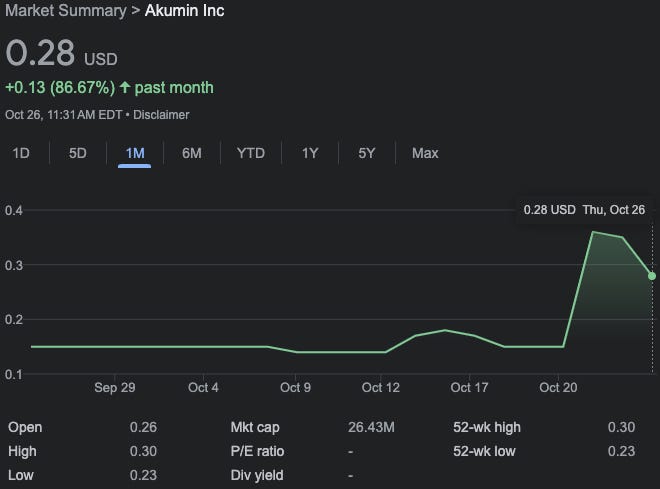This image displays a detailed market summary for AKUMIN, featuring various financial statistics and a performance graph for the past month. The top left corner contains a small grey text that reads "Market Summary," with a right-pointing arrow adjacent to it. In white text, prominently displayed is the name "AKUMIN," followed beneath in grey by the current stock price of "0.28 USD." 

Highlighted in green is the price change, "+0.13" (indicating growth), and the percentage increase, "86.67%," with an upward arrow beside it. Below this information, also in grey, is the timestamp "OCT 26 11:31 AM EDT," and a note marked as "DISCLAIMER."

Underneath these details is a horizontal selection bar, where "1D," "5D," and various other time interval options are listed in grey, except for "1M," which is in blue and underlined. This emphasizes that the data being viewed is for a one-month period. The intervals listed include "6M," "YTD," "1Y," "5Y," and "max," each separated by thin grey lines.

A grid chart beneath this bar shows the stock's daily closing prices over the month. The left axis is labeled with "0.04," "0.03," "0.02," and "0.01." The right axis at the top again lists "0.28 USD," with the date "THU, OCT 26" shown. The chart features a green line representing the stock's price movement: starting steady, dipping slightly, climbing, then soaring significantly before a minor decline.

Along the bottom of the graph are date markers: "SEP 29," "OCT 4," "OCT 9," "OCT 12," "OCT 17," and "OCT 20." Below the graph are additional financial metrics: 

- "OPEN: 0.26"
- "Market Cap: 26.43M"
- "52-WK HIGH: 0.30"
- "HIGH: 0.30"
- "P/E Ratio: -" 
- "52-WK LOW: 0.23"
- "LOW: 0.23"
- "Dividend Yield: -"

This provides a comprehensive snapshot of AKUMIN's stock performance and key financial data over the past month.